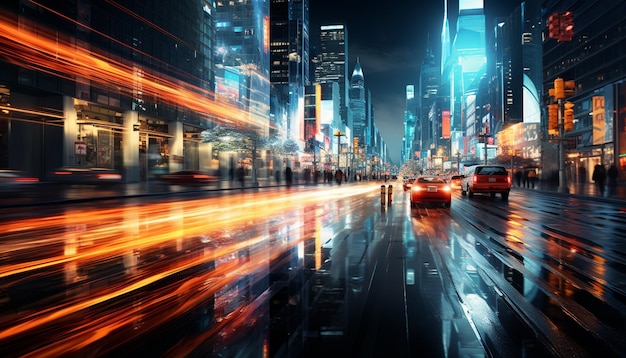This photo captures a vibrant, futuristic nighttime scene in a bustling downtown area, seemingly inspired by New York City. The image uses a time-lapse effect to accentuate the movement of lights, creating streams of orange light that shoot across the wet black street, suggesting the fast pace of city life. Skyscrapers dominate the skyline, their glowing façades illuminated in bluish-green hues, casting reflections on nearby buildings. Storefronts line both sides of the busy street, which features lanes of traffic moving in opposite directions—on the right, cars with brake lights on appear to be stopped at a light, while on the left, only streaks of headlights are visible. Blurred shapes of pedestrians populate the sidewalks, adding to the sense of motion. The scene is further animated by bright billboards, stoplights, and orange pylons. The dark gray, cloud-covered sky enhances the metropolitan ambiance, making the city feel alive and dynamic.